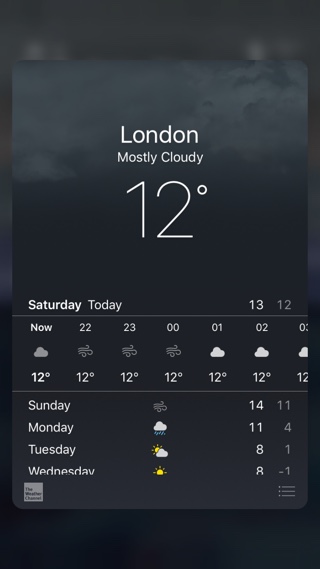A screen capture of a weather-related app with a dark background displaying a current forecast for London. The app indicates that it's mostly cloudy with a temperature of 12°C. The detailed hourly breakdown shows that from 10:00 PM to 3:00 AM, the weather will alternate between cloudy and windy, maintaining a steady temperature of 12°C. The extended forecast for the week is also provided: Sunday is expected to be windy with a temperature of 14°C, Monday will be cloudy at 11°C, Tuesday partly cloudy at 8°C, and Wednesday sunny at 8°C. At the bottom of the screen, the Weather Channel logo is prominently displayed.